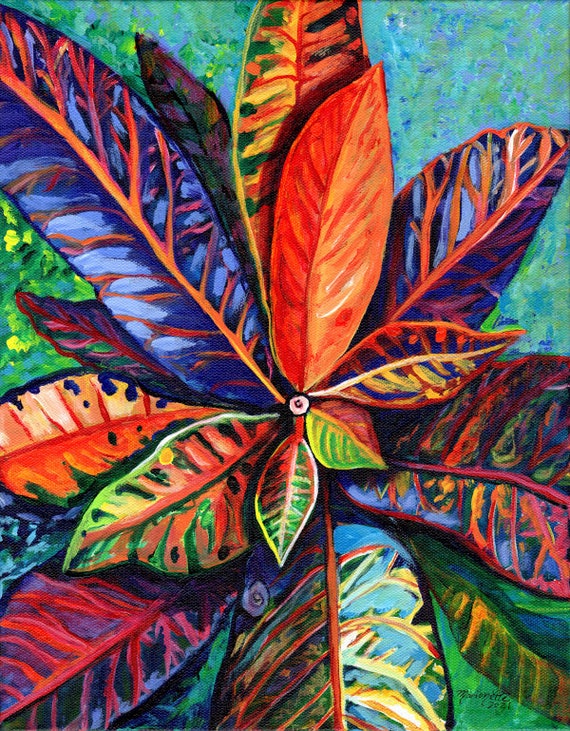This image is a detailed, abstract painting of a vibrant, flower-like plant. Rendered possibly in oil on canvas or digital medium, the composition captures a top-down perspective of the plant, radiating from a central point that resembles a small, white eyeball with a colorful center. The background is a soft blend of blue and green pastels, encasing the diverse array of vividly colored leaves that dominate the image.

The leaves, which vary in length and are narrow and pointy, are a dynamic mix of colors and patterns. There are multiple shades: solid bold blues, reds, and greens, as well as combinations featuring red veins on blue leaves, red and orange leaves interspersed with green, and spotted patterns. Each leaf is unique, contributing to the overall harmony of the painting's abstract nature.

The painting has a signed inscription in the bottom right corner, indicating its year, possibly 2001 or 2021, adding a hint of historical context to the piece.